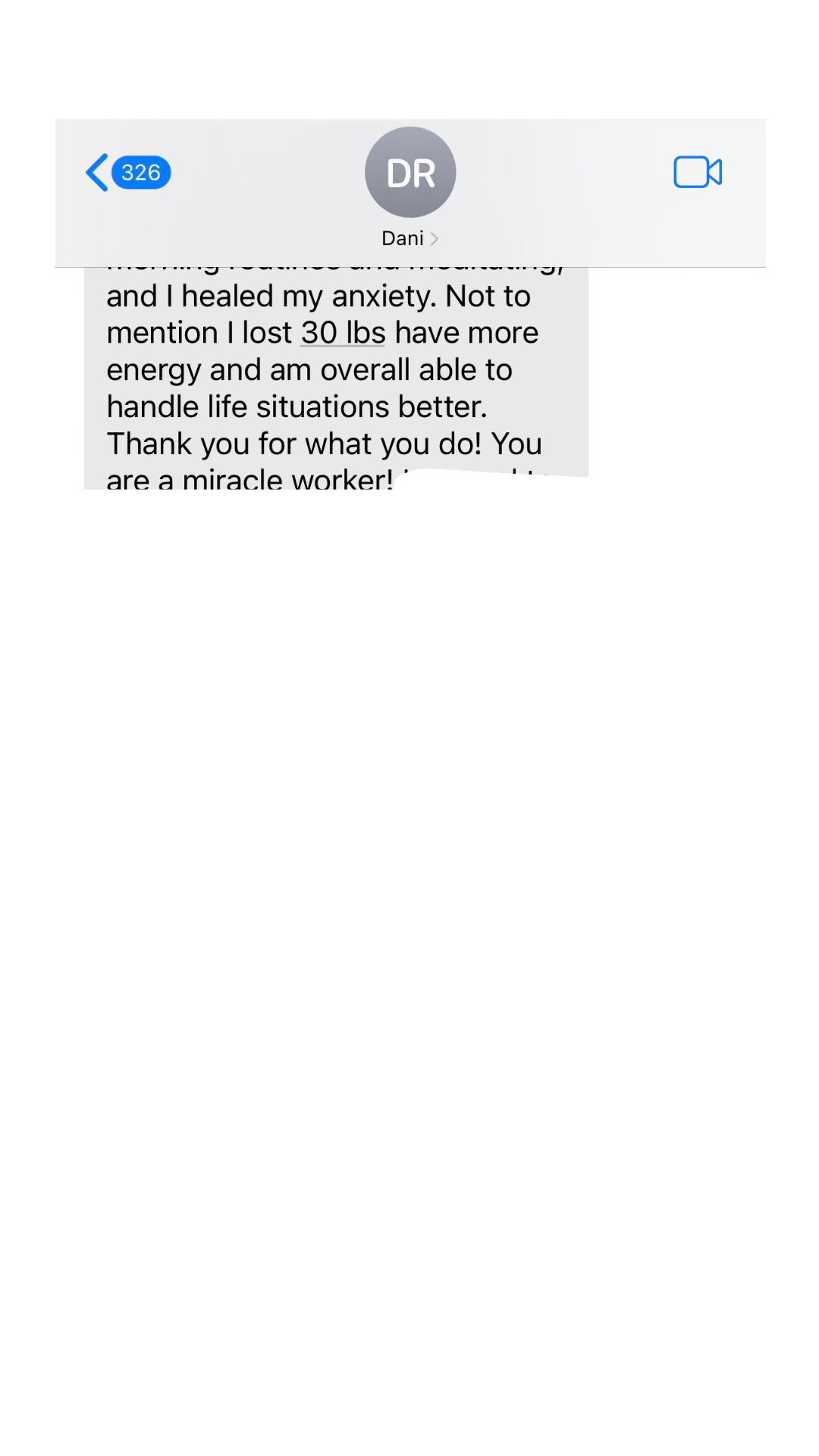This image is a cropped screenshot of a messaging application on an iPhone. At the top left, there's an icon resembling a blue pill with the number 326, likely indicating the count of unread messages. Adjacent to that is a "Back" button. To its right, there's an identifier for the phone's owner, displaying "DR" in capital letters inside a gray circle. Below this identifier is the name "Danny" followed by a right-facing arrow and the FaceTime logo, indicating an option to initiate a FaceTime call with Danny.

The main body of the message is set against a gray background with black text. The message reads: "And I heal my anxiety. Not to mention I lost 30 pounds. I have more energy. I'm overall able to handle life situations better. Thank you for what you do. You are a miracle worker." The area surrounding the gray background is white, providing contrast and clarity to the message.

In essence, this screenshot provides a view into a user's messaging interface, highlighting a testimonial message about personal improvements attributed to the recipient, Danny. The layout and design elements are typical of an iPhone messaging app, with the familiar FaceTime and message count icons.